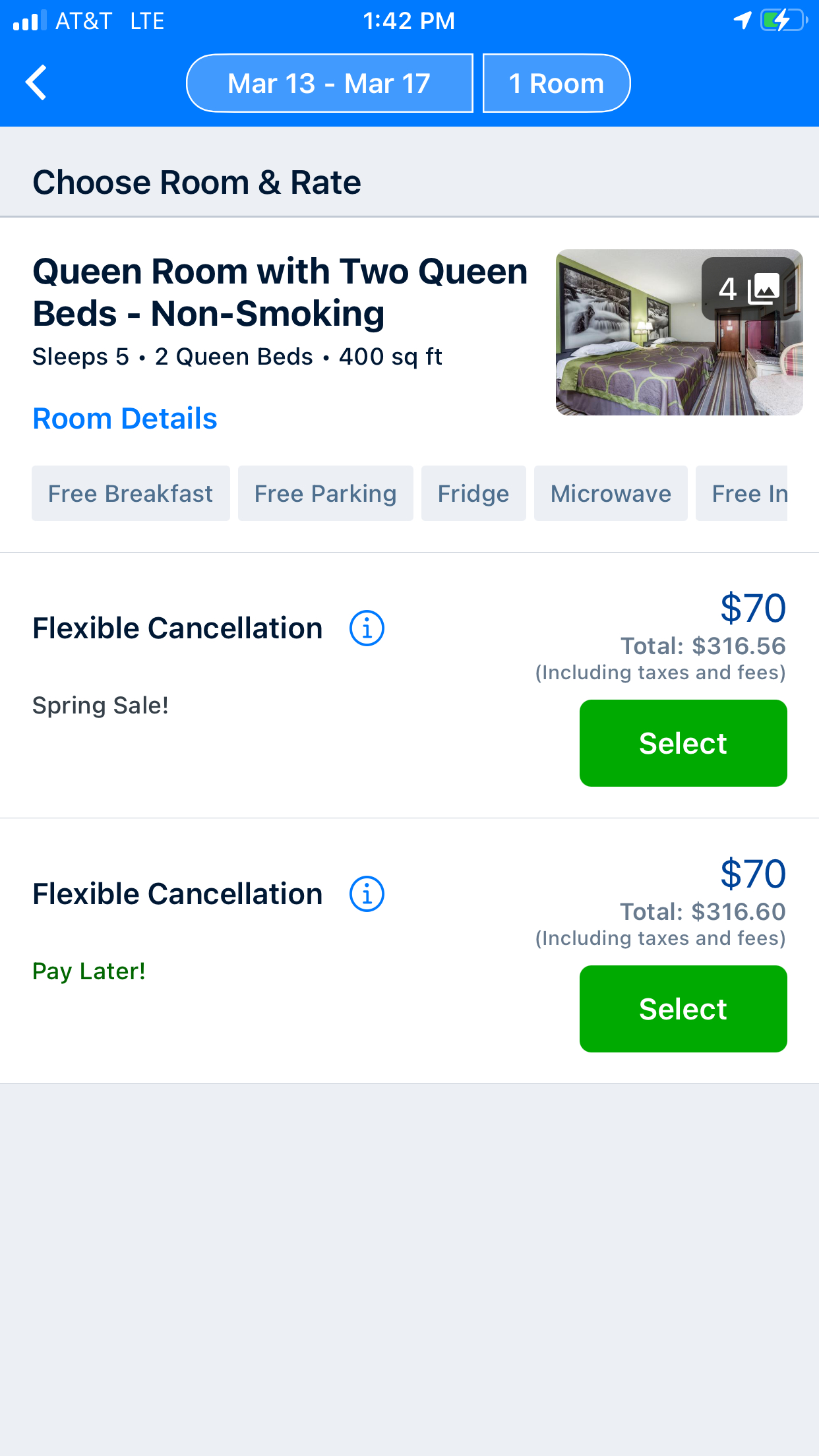This image displays a screenshot of a mobile-optimized website, likely for booking accommodations. At the top, a blue navigation bar with white text features essential mobile icons: four signal bars indicating AT&T LTE connectivity, the time stamped at 11:42 pm, a paper plane icon, and a half-full battery indicator on the right. Below this, a back arrow is visible alongside a central, curved rectangle displaying the text: "Mar 13 to Mar 17, one room." 

Further down, the screen transitions to a very light grey background with black text stating, "Choose room and rate." Below this, a white section presents details for a "Queen room with two queen beds, non-smoking," which can accommodate up to five guests within 400 square feet. This section mentions amenities such as free breakfast, free parking, fridge, microwave, although the text cuts off mid-sentence on the right side.

A room image is partially visible, showing a bed with a grey cover accented by green edges, and walls adorned with black and white pictures. The lighting seems to emit a yellow and green hue, and the walls are grey. A "4" icon suggests there are four images available for viewing. 

Continuing down, a thin grey line separates this section from additional booking details. Notable is a "Flexible cancellation" option marked by a blue information icon. Special pricing for a "Spring sale" is highlighted in blue, showing a rate of $70, with the total amounting to $316.56 including taxes and fees. A green "Select" button with white text is presented beneath this.

Following another thin horizontal line in black, further booking options reiterate the $70 pricing with a total of $316.80 including taxes and fees. Another "Flexible cancellation" line appears, paired with a blue information icon and a select button for booking. The phrase "Pay later" is visible under "Flexible cancellation," which appears under the "Spring sale" offer.

At the bottom of the screen, there is a grey rectangular box running the entire width of the website, leading down to a black section at the very bottom of the image.